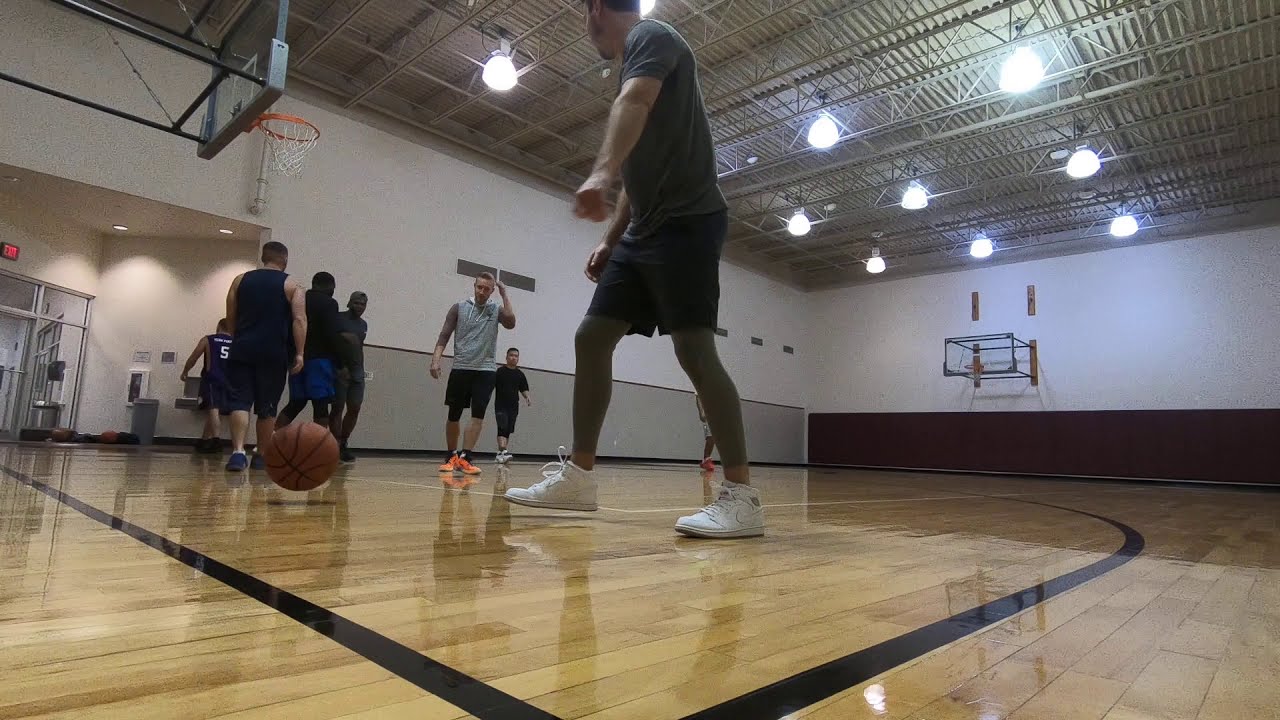The image captures a horizontally aligned rectangular photo of an indoor basketball gym at ground level. The gym's floor is a reflective, shined wood paneling marked with black lines outlining various areas of the basketball court. The far and closest walls feature gray-trimmed basketball hoops with see-through acrylic backboards and orange rims with white netting. The white-topped walls have gray and brown sections at the bottom. The gym is illuminated by hanging lights attached to a flat silver-gray ceiling. On the left side, there are windows and a glass exit door, beside which is a white fire extinguisher box with a red extinguisher, followed by a gray water fountain. In the middle of a game, about seven men are on the court. A basketball is in mid-bounce just above the ground. One central player, poised to pick up the ball, is dressed in white high-top shoes, leggings, blue shorts, and a gray t-shirt. Other players, also in shorts, are either walking away or towards the action, contributing to the dynamic scene.